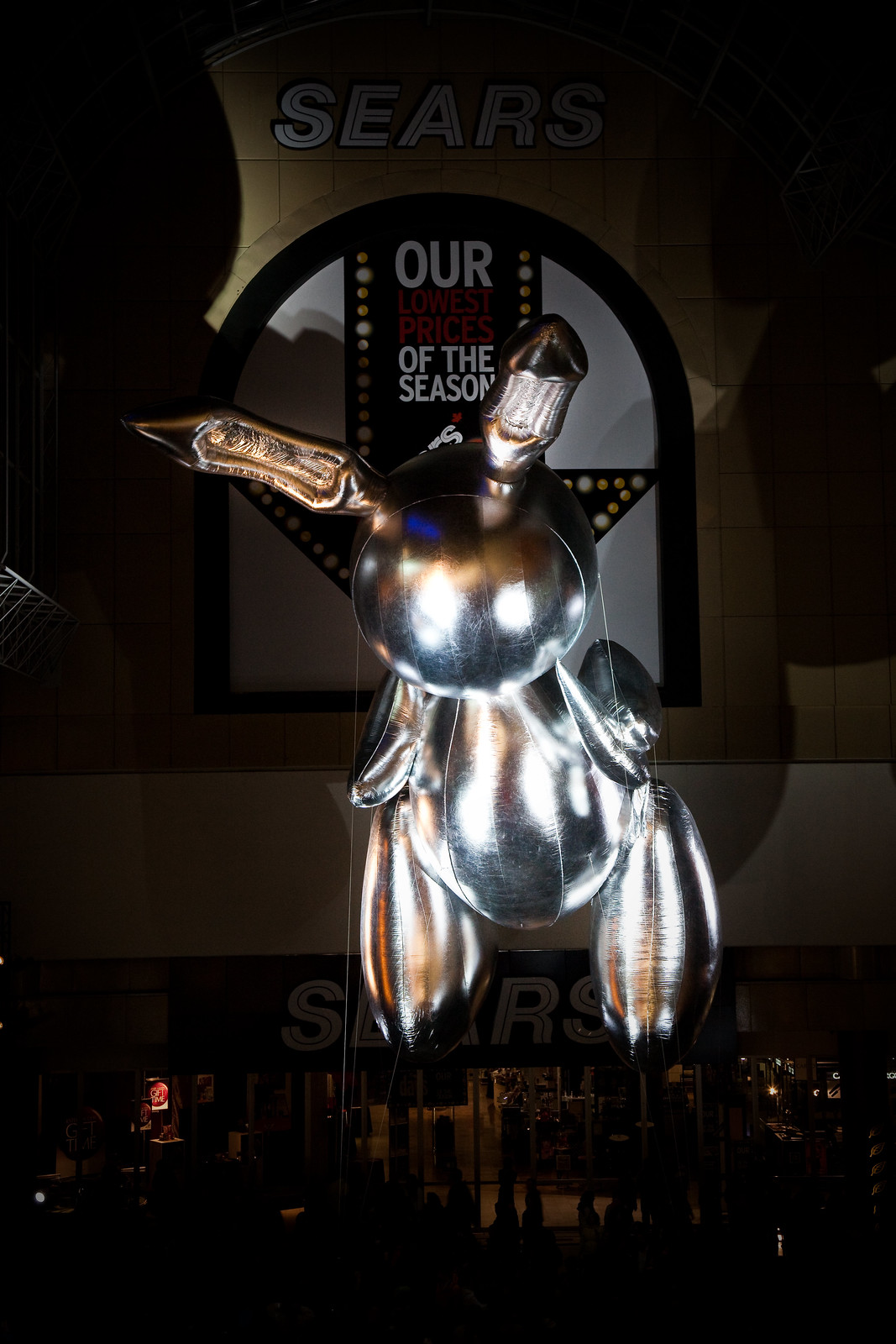The image depicts a large, silver sculpture or balloon with an ant-like appearance, prominently displayed in front of a Sears store at night. The sculpture has two bipedal legs with round feet, two round arms with small hands, a large round head, and two cylindrical ears extending from its head. It appears to be hovering or suspended in mid-air, illuminated by multiple lights. At the top of the image, a white sign reads "Sears," and beneath the sculpture, another partially obscured sign declares "our lowest prices of the season." Shadows of people can be seen below the sculpture, adding to the bustling nighttime ambiance. The store's glass storefront, including doors and windows, is visible at the bottom, offering a glimpse into the interior of the store.